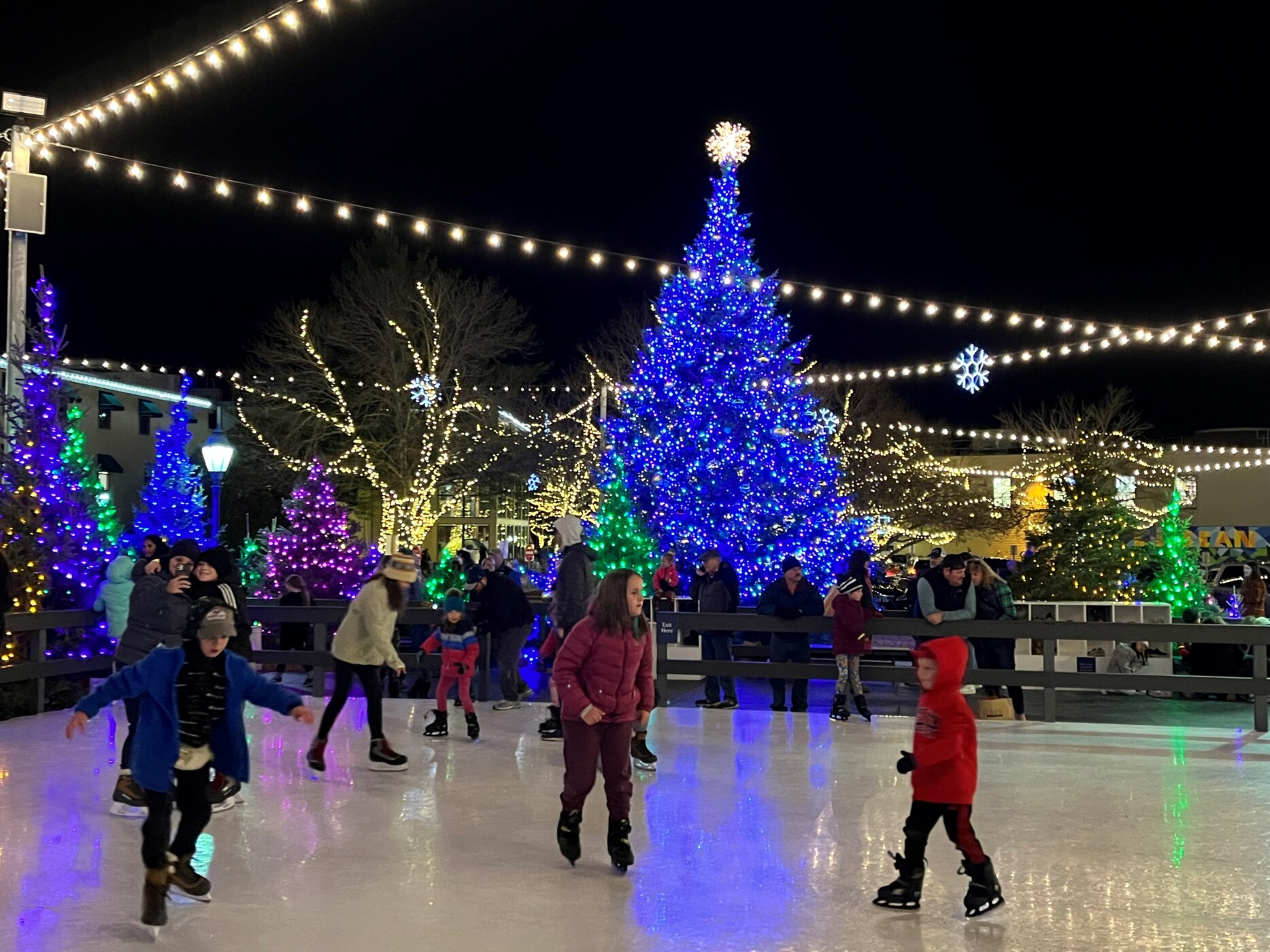In this detailed color photograph taken at night, a festive outdoor skating rink is set against the backdrop of a city park or public meeting place adorned with numerous Christmas decorations. The rink, encircled by a black or gray wooden fence, gleams with a shiny, reflective surface beneath a canopy of criss-crossing white string lights. Central to the scene is a large Christmas tree decorated in shades of purple, blue, and white, crowned with a white starburst at the top. Surrounding it are both natural trees adorned with white and yellow Christmas lights and smaller artificial trees in vibrant hues of purple, blue, and green. 

On the ice, around 10 to 15 skaters, both children and adults, glide gracefully, most donning hockey skates. Two women, bundled in warm winter jackets, pause on the left for a selfie amidst the cheerful atmosphere. Beyond the fence, spectators lean in to watch the skaters, bathed in the glow of festive lights. The dark night sky above and the outlines of nearby buildings frame this enchanting holiday scene, capturing the joyous spirit of the season.